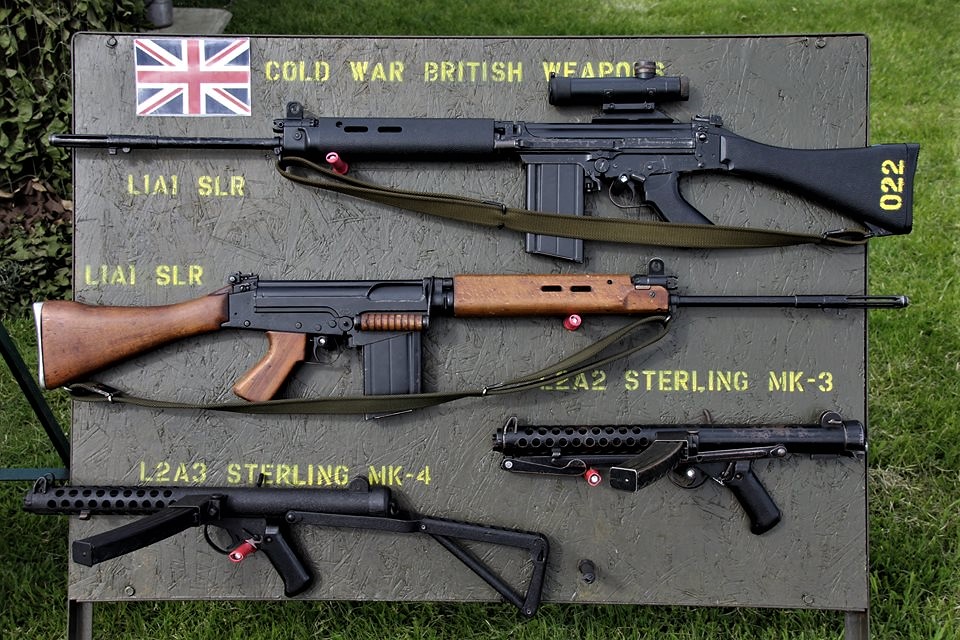The image depicts a display of four British firearms from the Cold War era mounted on a rectangular, dark gray metallic plaque with a striated surface, resembling rock facing. The title "COLD WAR BRITISH WEAPONS" is prominently displayed at the top of the plaque in gold uppercase font, accompanied by a small Union Jack in the upper left-hand corner. Each firearm is labeled in bold uppercase font.

The weapons are mounted in alternating directions: the top rifle is long and entirely black, marked with the number 022. The second firearm is a long rifle with a combination of black and wooden parts. Below these, two shorter, all-black guns are mounted; the third labeled as LEA-2 Sterling, and the fourth as LEA-3 Sterling, NIK-4. The plaque is supported by two metal legs, with grass visible in the background.